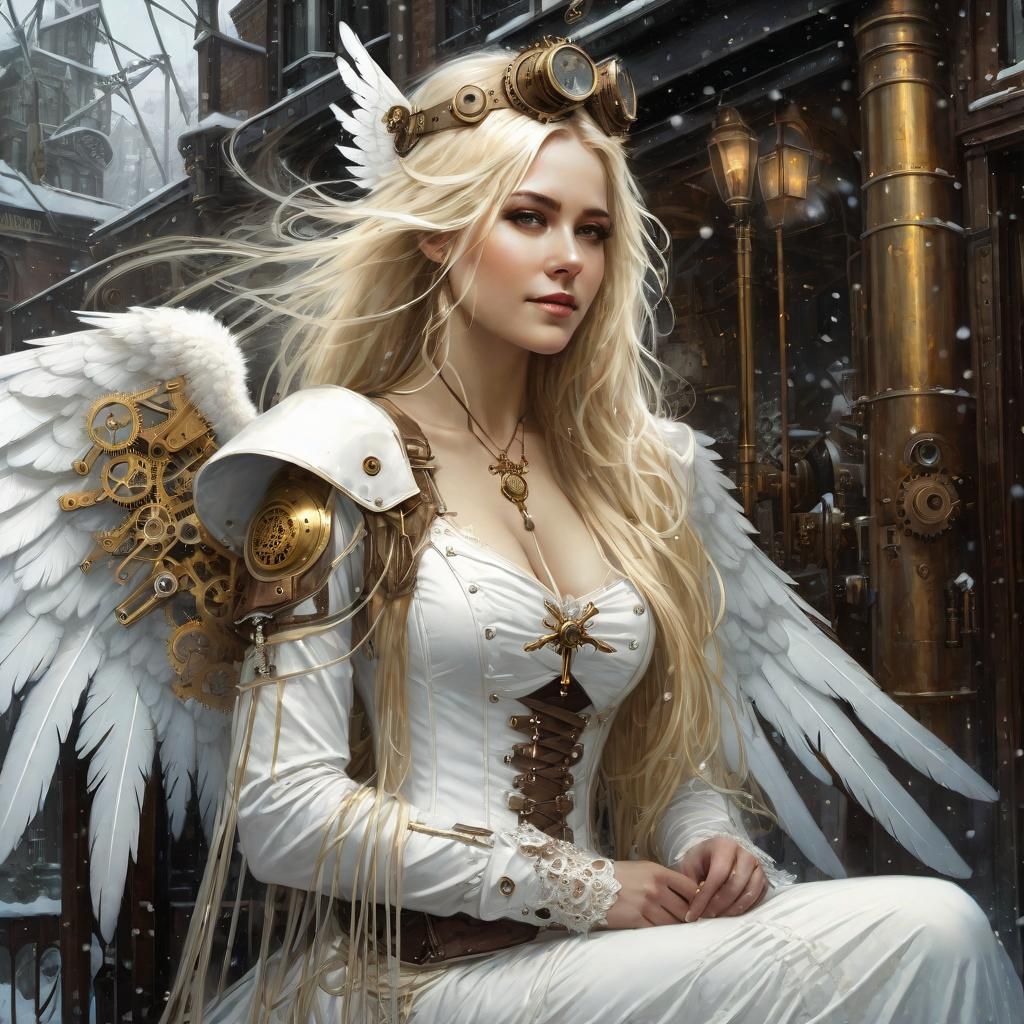The image depicts a highly detailed, realistic painting of a young blonde woman, possibly in her twenties, seated outdoors. She has long, wavy hair flowing past her waist, with some strands resting over her left shoulder and others seemingly blowing in the wind. She wears a white dress adorned with metallic embellishments and leather ties down the front, which also exposes some cleavage. A pendant, resembling a clock on a gold chain, dangles from her neck.

Perched atop her head is a pair of steampunk-style goggles made of bronze with glass lenses, and her left shoulder is protected by a piece of armor that combines both metallic and leather elements. Attached to her back are large, spread-out white wings with detailed feathers and mechanical elements featuring gears, giving them a robotic appearance.

The setting is steampunk-themed, with copper pipes, lampposts with golden hues, and speckles in the air that could be snow. The background includes tall metal structures and buildings, one with a fire escape and another cylindrical structure with gears, contributing to the overall metallic and futuristic ambiance. The woman, who has a neutral expression and looks directly at the viewer, rests her hands on her lap, completing the serene yet complex scene.